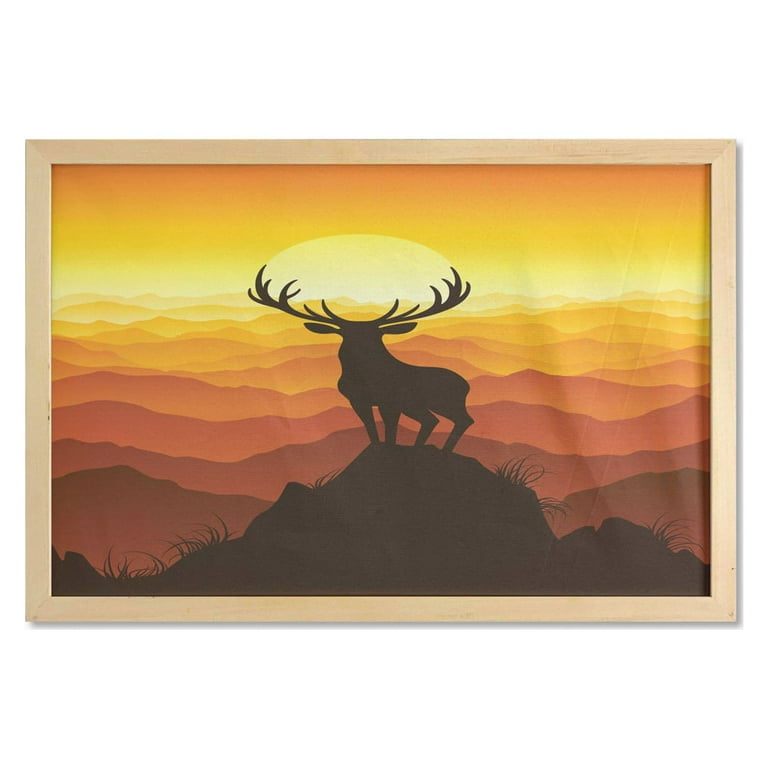The image depicts a rectangular artwork, encased in a light brown wooden frame. The centerpiece of the artwork is the silhouette of a male buck with large horns, standing poised on a rocky outcrop adorned with patches of grass. The backdrop features a harmonious gradient of colors, transitioning from dark red at the bottom to orange, yellow, and white, and then back to orange at the top. Behind the deer, rolling ridges or mountain tops extend in varying shades of brown, orange, gold, and yellow, leading up to a setting sun. The sun, a blend of light yellow and white, appears as a half circle on the horizon, casting a serene glow on the scene. The overall style of the image has a simplistic, vector art aesthetic, set against a predominantly solid white background that accentuates the vivid colors of the artwork.